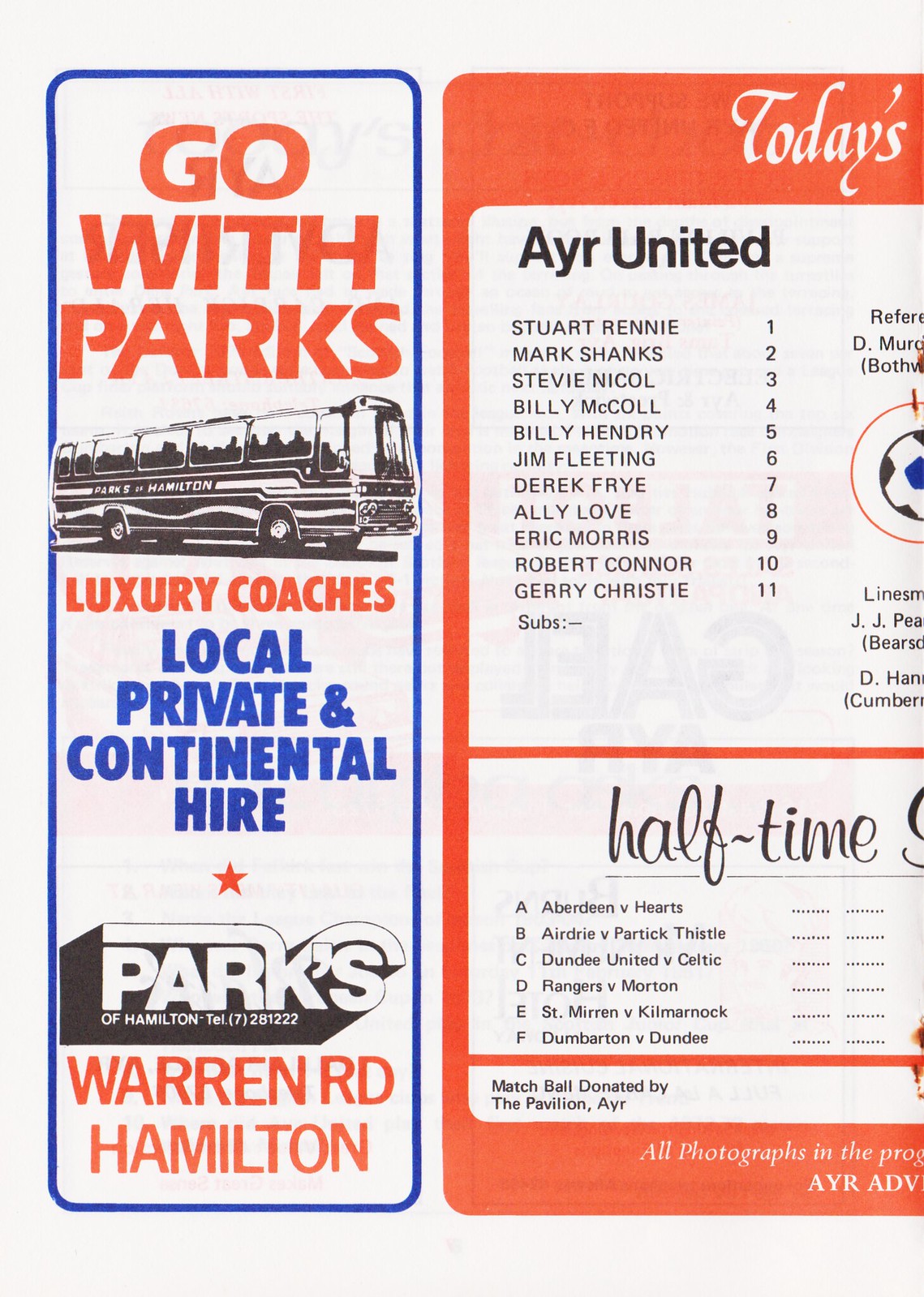This image appears to be a page from a sports program, likely detailing a soccer match schedule for Ayr United. On the left-hand side of the page is an advertisement for Parks of Hamilton, a luxury coach service. The ad features a bold red tagline that reads "Go with Parks," followed by a black and white illustration of a coach-style bus labeled "Parks of Hamilton" with silhouettes of people visible through the windows. Below the bus, red text announces "Luxury Coaches," and blue text lists services offered: "Local, Private, and Continental Hire." Further down, a red star is displayed, accompanied by the company's name and address, "Parks of Hamilton, L7281222, Warren Road, Hamilton," outlined in blue.

On the right-hand side, partially visible behind the ad, is a match day schedule. It begins with the partially cut-off heading "Today's" in orange-red text, followed by what remains of the title "Ayr United" in black lettering on a white background. The player roster for Ayr United is listed: Stuart Runny, Mark Shanks, Stevie Nichol, Billy Nicole, Billy Hendry, Jim Fleeting, Derek Fry, Allie Love, Eric Morris, Robert Conner, and Gary Christie. There are no substitutes listed. Additional details include referee names and possibly linesmen, with sections marked for halftime activities. Other club matches mentioned include Aberdeen versus Hearts and Dundee United versus Castle. The bottom of the page notes the match ball donation by the Pavilion Air and indicates that all photographs are found in the program.